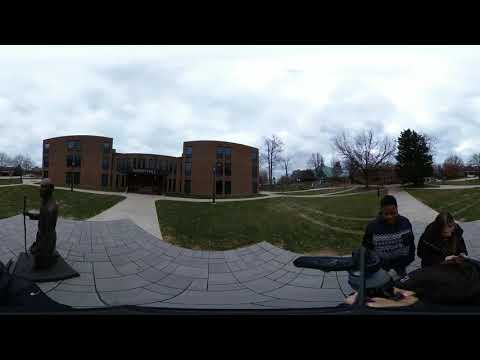The image depicts an outdoor scene likely taken in the middle of the day in front of a school. The photograph is framed by a solid black border at the top and bottom. At the bottom left, a statue stands on a concrete tile, while in the bottom right, two individuals are visible. The person on the left, identified as a black man, wears a black and white sweater and has tan skin. The person on the right, a woman with long brown hair and fair skin, wears a black coat. They appear to be standing and looking at something on a stand in front of them.

The central area of the image is dominated by a large expanse of grass, intersected by a gray concrete pathway leading up to a large brown building situated slightly to the top left of the center. This building appears to be part of a school complex, featuring two distinct hemispheres. Surrounding the building are trees, bushes, and additional houses. The sky above is overcast with clouds, casting a subdued light over the scene. The colors in the image include black, white, gray, brown, light gray, green, and tan, creating a muted yet detailed landscape.